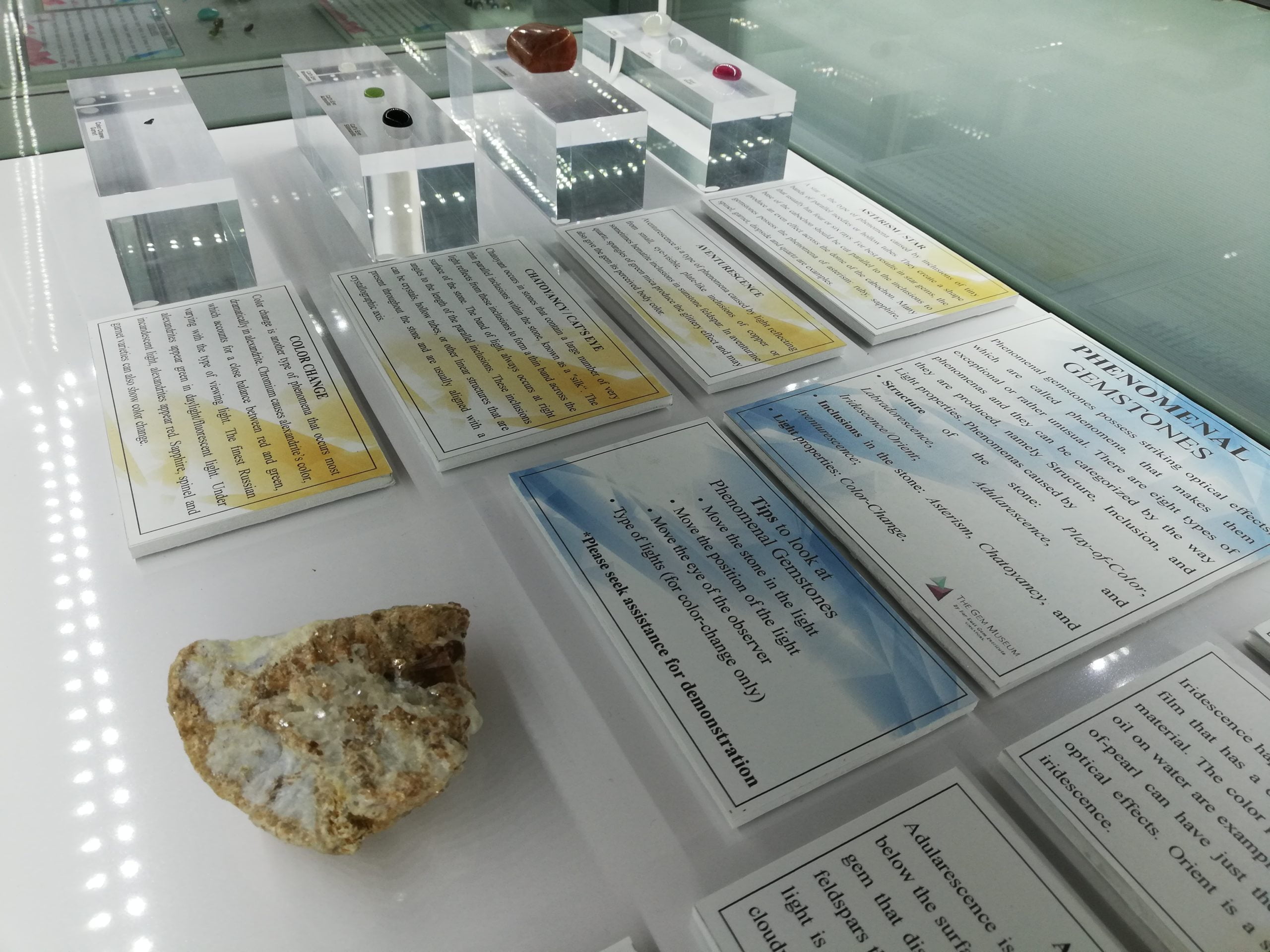The image presents a detailed view of a museum exhibit showcasing gemstones, likely in a natural history museum. The perspective runs down a long display case resembling a clear-topped table often seen in jewelry stores. The case stretches away from us, with its white base supporting various raised plaques and gemstones. At the forefront, to the left, sits a large, reflective gemstone exhibiting hues of cream, brown, tan, and gray with diamond-like shiny flakes. Above this prominent gemstone, a blue-and-white sign reads "Phenomenal Gemstones," followed by descriptive text about the exhibit. The initial row features four lofty glass platforms displaying gemstones, higher than the subsequent plaques. The second row comprises four plaques with a yellow accent, while the third row includes two plaques with a blue accent, alongside a base-positioned gemstone. In the lower right corner, another barely visible row of plaques suggests more information. Additional smaller rock displays on stands are faintly discernable in the background.